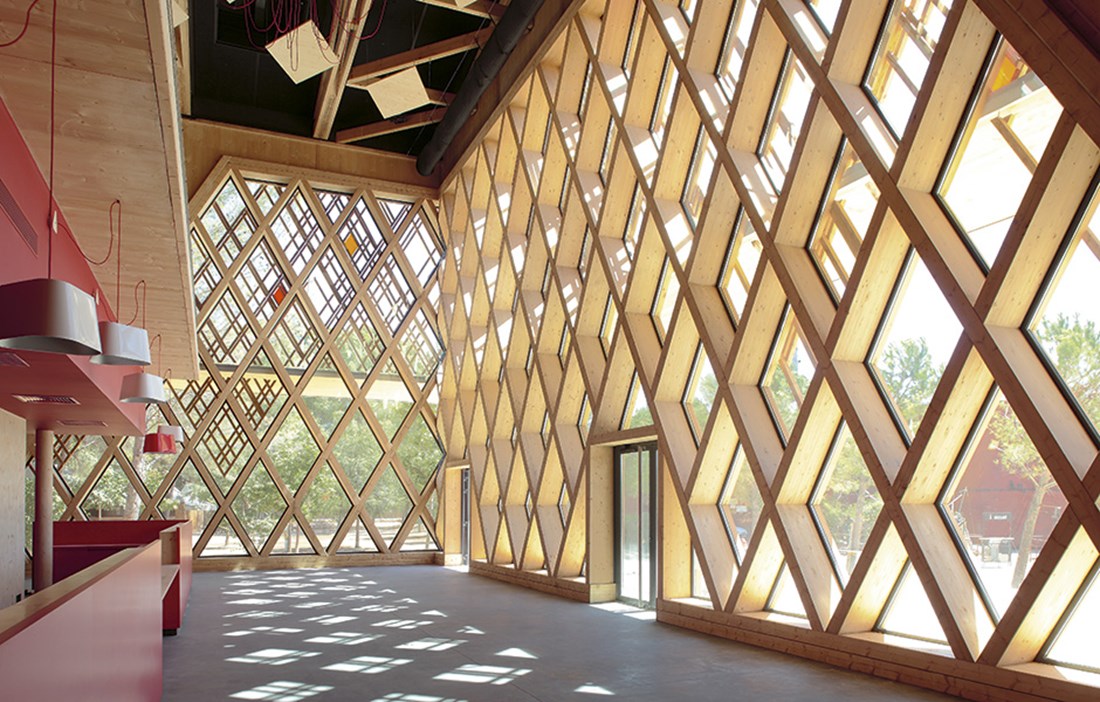This image showcases a large indoor room that feels almost outdoors due to the abundance of natural light pouring in through numerous diamond-shaped windows. These floor-to-ceiling windows, framed by light beige wooden borders, form a striking gold crisscross design that extends along the entire right wall and continues to the back wall. The floor is a gray marble or cement with dark gray shadows cast by the sunlight.

In the left section of the room, there's a red counter with a light wooden top, situated beneath a wooden awning. Hanging from the awning are lamps with white lampshades. The ceiling features recessed lighting in the upper left corner. Outside the diamond-shaped windows, a red building is visible in the lower right corner, and an orchard-like scene with numerous trees is seen in the center-left, enhancing the room's open and airy atmosphere.